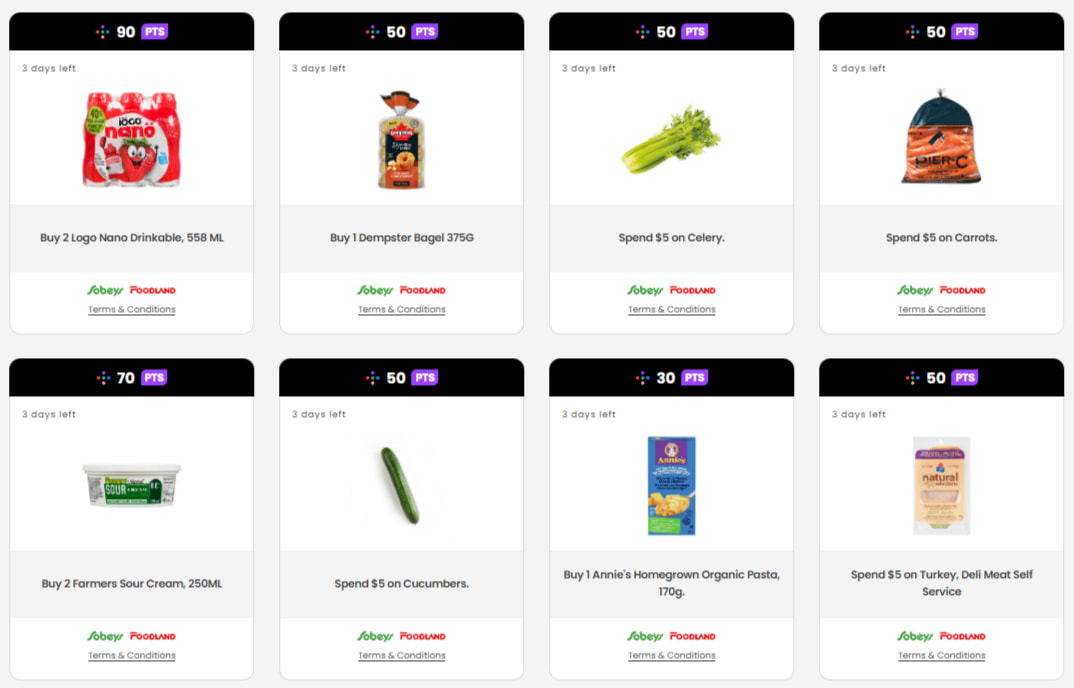**Image Description:**

The image appears to be a promotional grid layout from a shopping site. The overall design features a light gray border approximately a quarter of an inch thick that frames the entire image. Inside this frame, the layout is divided into two rows, each containing four rectangular sections, making a total of eight sections.

Each rectangle has a gray border separating it from the others, with additional horizontal and vertical gray lines delineating each section further. The top border of each rectangle is black and includes a white number indicating point values.

**Top Row:**

1. **First Rectangle:**
   - **Top Black Bar:** 90 PTS
   - **Left Corner:** "3 days left" (white background)
   - **Image:** A product image
   - **Gray Border Label:** BATU Logo Nano Drinks 558 ML
   - **Additional Labels:** 
     - "Phobies" (green text on white background)
     - "Foodland" (red text)
   - **Underline:** "Terms and Conditions" (black, underlined)

2. **Second Rectangle:**
   - **Top Black Bar:** 50 PTS
   - **Left Corner:** "3 days left" (white background)
   - **Image:** Dempster Bagel
   - **Gray Border Label:** Buy One Dempster Bagel 375G
   - **Additional Labels:** 
     - "Phobies" (green text on white background)
     - "Foodland" (red text)
   - **Underline:** "Terms and Conditions" (black, underlined)

3. **Third Rectangle:**
   - **Top Black Bar:** 50 PTS
   - **Left Corner:** "3 days left" (white background)
   - **Image:** Celery
   - **Gray Border Label:** Spend $5 on Celery
   - **Additional Labels:** 
     - "Phobies" (green text on white background)
     - "Foodland" (red text)
   - **Underline:** "Terms and Conditions" (black, underlined)

4. **Fourth Rectangle:**
   - **Top Black Bar:** 50 PTS
   - **Left Corner:** "3 days left" (white background)
   - **Image:** Carrots
   - **Gray Border Label:** Spend $5 on Carrots
   - **Additional Labels:** 
     - "Phobies" (green text on white background)
     - "Foodland" (red text)
   - **Underline:** "Terms and Conditions" (black, underlined)

**Bottom Row:**

1. **First Rectangle:**
   - **Top Black Bar:** 70 PTS
   - **Left Corner:** "3 days left" (white background)
   - **Image:** Sour Cream
   - **Gray Border Label:** BATU Farmer Sour Cream 250 ML
   - **Additional Labels:** 
     - "Phobies" (green text on white background)
     - "Foodland" (red text)
   - **Underline:** "Terms and Conditions" (black, underlined)

2. **Second Rectangle:**
   - **Top Black Bar:** 50 PTS
   - **Left Corner:** "3 days left" (white background)
   - **Image:** Cucumber
   - **Gray Border Label:** Spend $5 on Cucumbers
   - **Additional Labels:** 
     - "Phobies" (green text on white background)
     - "Foodland" (red text)
   - **Underline:** "Terms and Conditions" (black, underlined)

3. **Third Rectangle:**
   - **Top Black Bar:** 30 PTS
   - **Left Corner:** "3 days left" (white background)
   - **Image:** Annie's Homegrown Organic Cosmo
   - **Gray Border Label:** Buy One Annie's Homegrown Organic Cosmo 170 Grams
   - **Additional Labels:** 
     - "Phobies" (green text on white background)
     - "Foodland" (red text)
   - **Underline:** "Terms and Conditions" (black, underlined)

4. **Fourth Rectangle:**
   - **Top Black Bar:** 50 PTS
   - **Left Corner:** "3 days left" (white background)
   - **Image:** Turkey in Plastic Packaging
   - **Gray Border Label:** Spend $5 on Turkey, Deli Meats Self-Service
   - **Additional Labels:** 
     - "Phobies" (green text on white background)
     - "Foodland" (red text)
   - **Underline:** "Terms and Conditions" (black, underlined)

The layout is consistent in formatting, with variations in point values and product descriptions, indicating different promotions for various items.